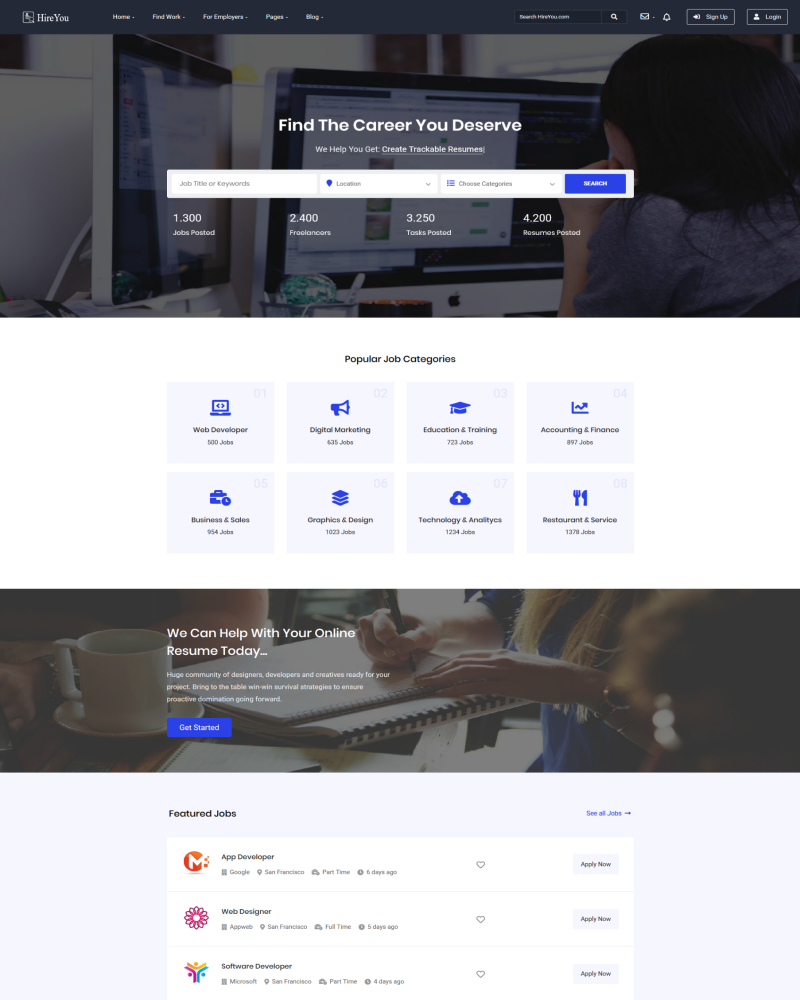This screen capture depicts the homepage of a job search website predominantly designed in dark gray and black tones. At the very top, a sleek black header bar displays the site name "Hire You" in white text. To the right, a white menu extends across the dark background, listing options such as Home, Find Work, For Employers, Pages, and Blog. On the far right of this bar, a search field is flanked by an envelope icon, a notification bell, a Sign Up button, and a Login button.

The central image features a shadowy figure on the right side, intently staring at two computer monitors situated on the left. Across the monitors, the bold white text reads, "Find the Career You Deserve. We Help You Get, Create, Trackable Resumes." Below this motivational message, a white bar includes fields for entering a Job Title or Keywords, Location, and Choose Categories, with a prominent blue search button on the right.

Statistics listed on the site highlight its scope and activity: 1,300 jobs posted, 2,400 freelancers, 3,250 tasks posted, and 4,200 resumes posted. Popular job categories are displayed beneath, including Web Developer, Digital Marketing, Education and Training, Accounting and Finance, Restaurant Service, Technology Analytics, Graphics Design, and Business and Sales.

Further down, another dark-themed image mirrors the top's aesthetic, accompanied by the text, "We can help you with your online resume today." At the very bottom, a section titled Featured Jobs showcases listings for positions such as App Developer, Web Developer, and Software Developer.